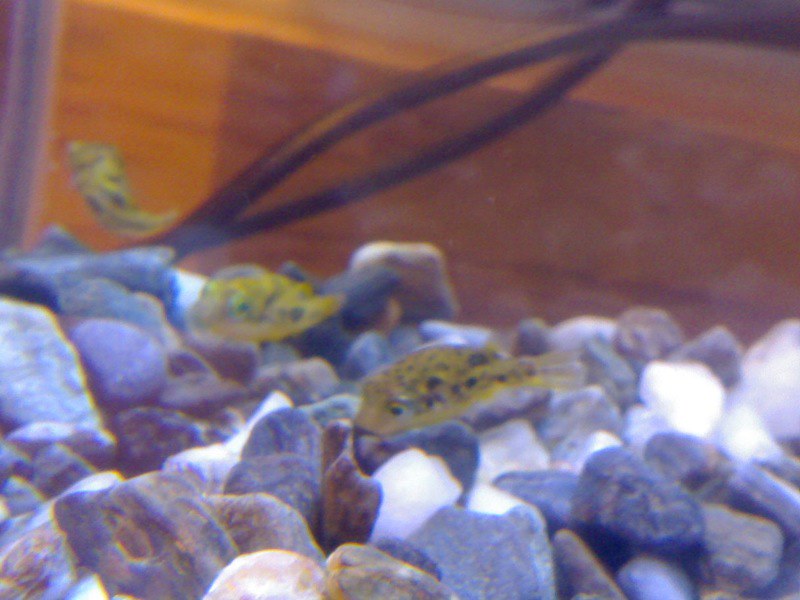This image is a close-up shot of an aquarium, taken indoors with a regular camera. The photograph is somewhat blurry, likely due to the zoom and the presence of plexiglass and water. The focus is on three fish, prominently colored yellow with black markings, though one fish on the far right has an orange, opaque hue with black spots. The tank contains no plants or greenery, just an array of multicolored rocks in shades of white, gray, dark blue, purple-burgundy, and some hints of orange. Visible in the background is a wire likely for the tank's filter and light, and behind the tank is a wooden surface that could be a piece of furniture or a wall, adding to the indoor setting.